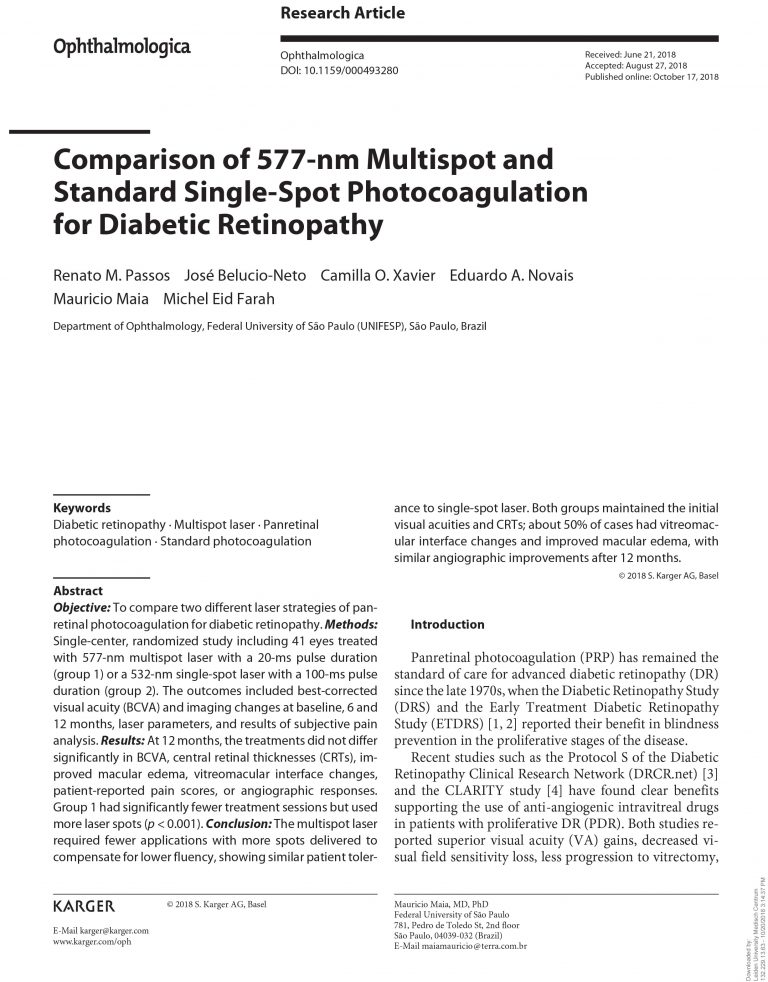The image is of the title page of a research article labeled "Research Article" at the top. The article is from the Department of Ophthalmology at the Federal University of Sao Paulo, Brazil, and was published in a journal associated with Ophthalmologica. The title of the article is "Comparison of 577-NM Multi-Spot and Standard Single-Spot Photocoagulation for Diabetic Retinopathy." Contributing authors are Renato M. Passos, Jose Belluccio Neto, Camila O. Xavier, Eduardo A. Novias, Mauricio Maia, and Michael Eid-Ferra. The article includes keywords such as diabetic retinopathy, multi-spot laser, pan-retinal photocoagulation, and standard photocoagulation, highlighting the focus on comparing two laser strategies for treating diabetic retinopathy. Additional details on the page include the DOI number, and information about the article being received on June 21, 2018, accepted on August 27, 2018, and published online on October 17, 2018. The abstract and the top part of the introduction are also visible, with the introduction mentioning "pan-retinal photocoagulation (PRP)." The page features a primarily black and white layout typical of academic publications, and at the bottom, the journal's name "Karger" is printed.